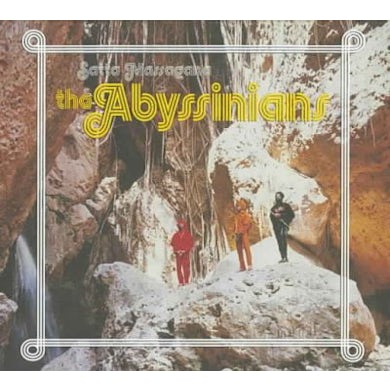The album cover features a color photograph of what appears to be the interior of a cavern or large crevice, bathed in sunlight streaming from above. At the forefront, a towering rock formation dominates the scene, crowned by a cascading waterfall and surrounded by an abundance of stalactites or hanging roots. Three band members stand atop this rock, their distinct outfits adding a splash of color against the natural backdrop: the central figure in a striking red jumpsuit, the member to the right in an orange jumpsuit, and the one on the far right in black attire. The overall design is encased within a meticulously crafted white border, formed by intertwined lines that loop into circles at the corners.

Above the band members, the album title is prominently displayed; the larger text in vibrant yellow font spells out "The Abyssinians" in artistic lettering, and above it, in smaller, hard-to-read white letters, "Sata Masagana". The cover, with its perfect square shape, conveys a strong vintage aesthetic reminiscent of the 1970s era, enhanced by the cohesive blend of natural and abstract elements in both the image and typography.